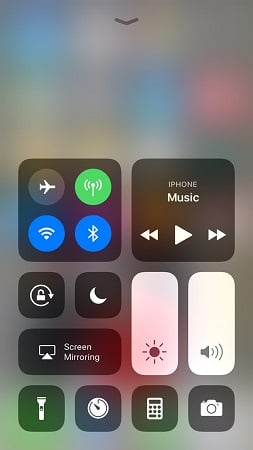The image appears to be a screenshot of a smartphone's control center in lock mode. The background is a gray overlay, rendering the icons of various applications grayed out and partially visible. Dominating the scene is an array of control icons, each distinctly colored and symbolized.

In the upper portion, there is a gray airplane symbol indicating that Airplane Mode is off. Adjacent to it, a green symbol that looks like a stick with a circle on top and two lines on either side likely represents active mobile data or a specific status indicator. 

Below these icons, the familiar Wi-Fi signal is prominently displayed in blue, indicating that the device is connected to a Wi-Fi network. Next to it is a blue Bluetooth symbol, showing that Bluetooth is enabled.

The control center also includes a section for media playback under "iPhone Music," with corresponding controls. A brightness control is depicted by a white rectangle with a sun icon, indicating that the screen brightness is set to maximum. Similarly, the volume control, represented by a speakerphone icon, is also maximized.

Additional shortcuts include icons for a flashlight, a calculator, and a camera, facilitating quick access to these functions directly from the lock screen.